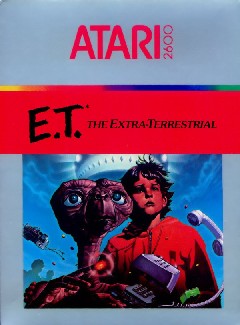This image appears to be from the early 1980s, featuring the box art for an Atari 2600 game. Prominently displayed at the top is "Atari 2600" in bold lettering. Below that, in the center, "E.T. the Extraterrestrial" is written in black letters against a striking red background. The artwork beneath this title is a detailed illustration rather than a photograph. It depicts E.T. and a young boy standing together, with an old-fashioned rotary telephone placed nearby. In the backdrop, a spaceship can be subtly seen amidst the trees, adding an element of mystery. The boy is dressed in a bright red shirt, while E.T. is illustrated in a reddish-brown hue. There are also a couple of human figures slightly visible among the trees, adding depth to the scene.